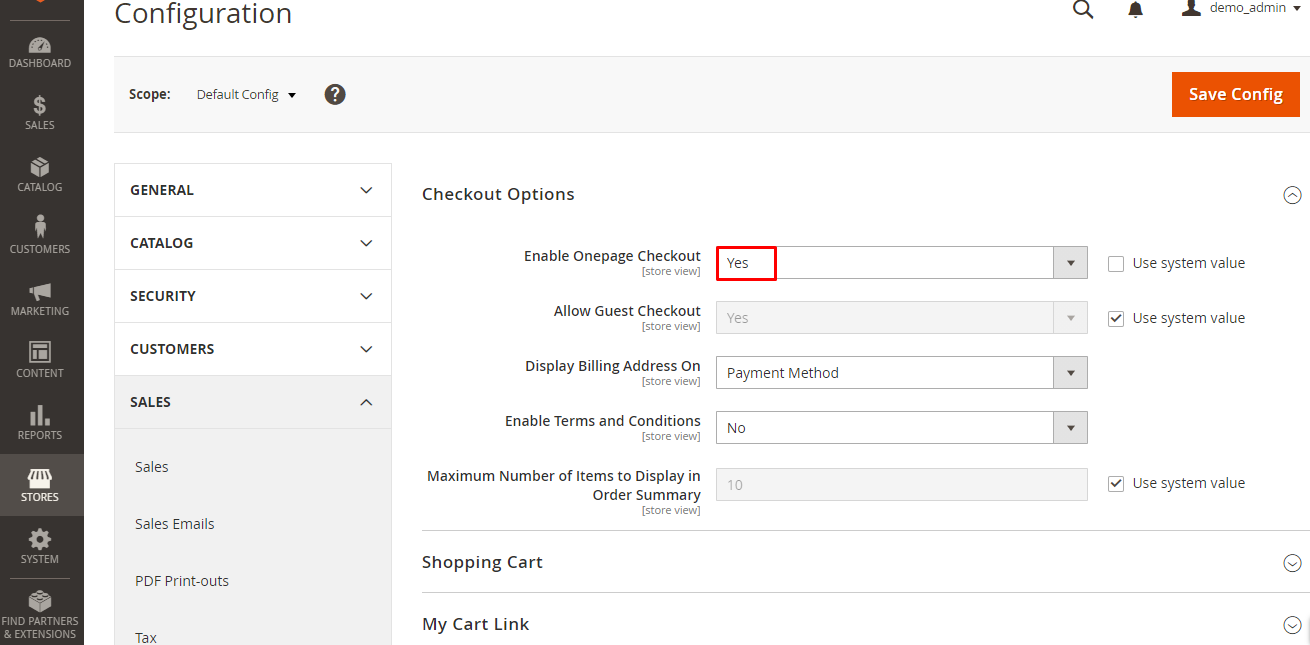This image depicts a web page displayed on a computer monitor for configuration purposes. At the top of the page, there are several icons and elements aligned from left to right: a search icon, a notification icon, a user icon, the text "demo_admin," and a dropdown arrow.

The left side of the screen features a black vertical sidebar listing various sections, including Dashboard, Sales, Catalog, Customers, Marketing, Content, Reports, Stores, System, and Find Partners and Extensions.

Just to the right of this sidebar, there is a light gray vertical bar. At the top of this bar, 'Scope' is indicated on the left side, with 'Default Config' and a dropdown arrow next to it. Further to the right in the same bar is a black circle containing a question mark icon, and at the far right, there is an orange 'Save Configuration' button.

Below this area, a series of sections with dropdown arrows are listed: General, Vertical, Catalog, Security, Customers, with the 'Sales' section expanded. This expanded section, which is a slightly darker gray, includes categories such as Sales, Sales Emails, PDF Printouts, and Tax.

The main body of the page displays a 'Checkout Options' section. Here, you can enable or disable various checkout settings. The 'Enable One-Page Checkout' option is controlled by a dropdown, currently set to 'Yes' within a red box. Additional checkout settings include 'Allow Guest Checkout' and 'Display Billing Address On Payment Method,' each with dropdown arrows for selection. Another option is 'Enable Terms and Conditions,' which is set to 'No' and also features a dropdown arrow. The 'Maximum Number of Items to Display in Order Summary' is set to 10 and marked with 'Use System Value.'

Underneath this checkout section is a light gray line separating it from the 'Shopping Cart' section, which includes dropdown arrows for 'Shopping Cart' and 'My Cart Link' options.